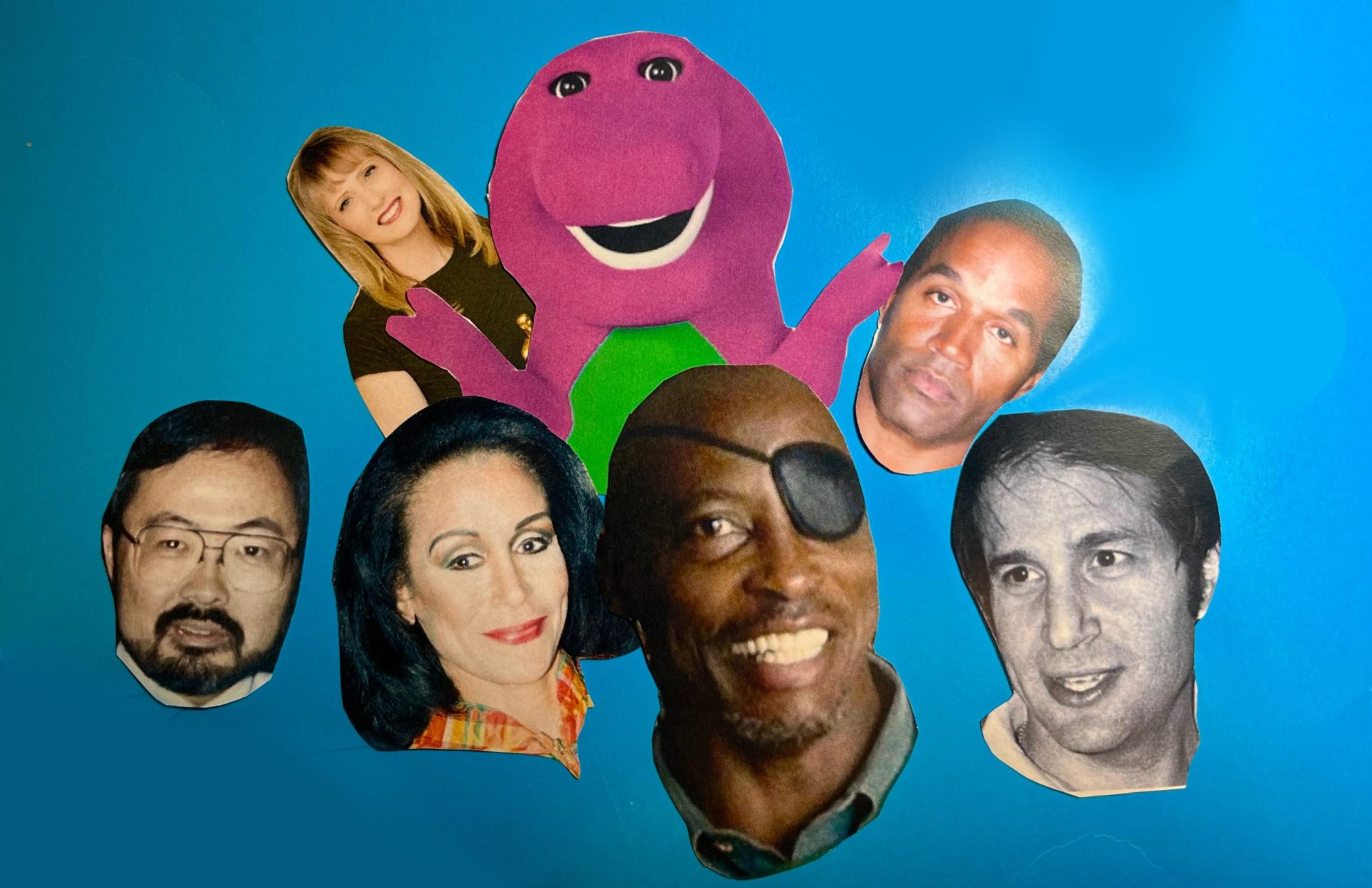In this detailed collage against a blue background, at the center is the iconic 1990s kids' character, Barney the Dinosaur, recognizable by his purple body and green tummy. His arms are extended, and notably, his face is replaced with that of O.J. Simpson. Surrounding Barney are various other famous and unrecognized faces. To Barney's right (viewer's left) is a blonde woman with chest-length hair and bangs. Adjacent to her is a black and white image that is difficult to identify. To Barney's left (viewer's right) is another cutout of O.J. Simpson's face, followed by a woman with shoulder-length black hair and an orange and red shirt collar, who appears of potential Middle Eastern descent. Below this array, in the front row, is an Asian man with a beard, mustache, and glasses, and next to him, seemingly judge Lance Ito from the O.J. Simpson case. Centered but lower is a smiling black man, identified as Wesley Snipes, distinguished by his black eye patch. Finally, to the right of Wesley Snipes is a white man with black hair. The composition is a vibrant and eclectic mix that highlights various recognizable figures and some whose identities aren't immediately clear.